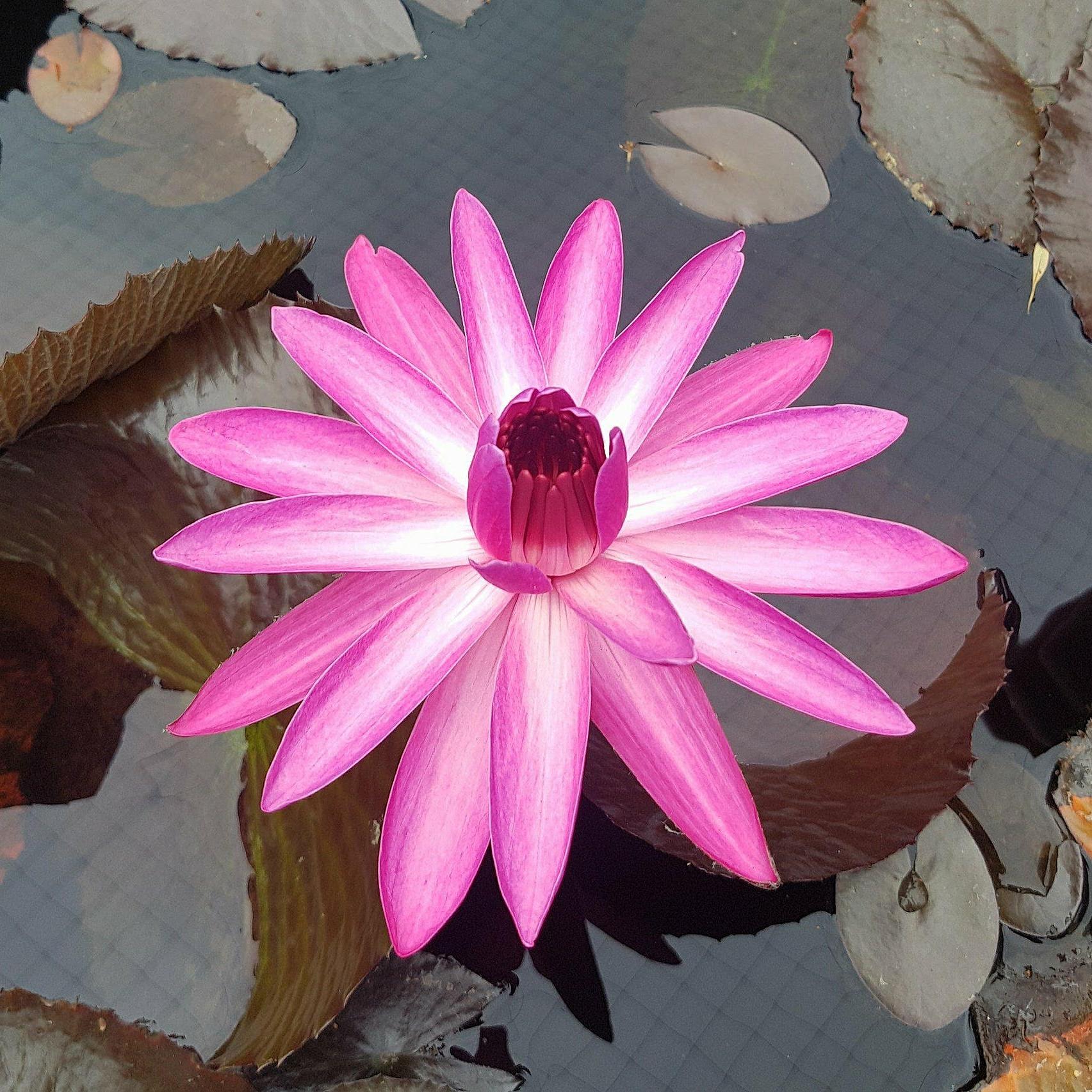The image is a detailed artwork, possibly a painting or a drawing, showcasing a vibrant pink lotus flower seen from nearly a top view. The lotus, which contrasts starkly with the mostly muted background colors, features numerous petals organized in several layers. The outer layers are open, revealing inner layers that are just beginning to bloom. The petals have a gradation from pink to white towards the top. Surrounding the vivid lotus, which commands the center of the image, the artwork is imbued with various muted shades, including pale blue, gray, brown, and hints of yellow and orange. In the background, one can discern details such as brown mushrooms and a checkered board pattern in blue, adding texture and complexity to the scene. The water surface behind the flower bears lotus leaves that are tinted gray or brown, enhancing the tranquil yet intricate composition.